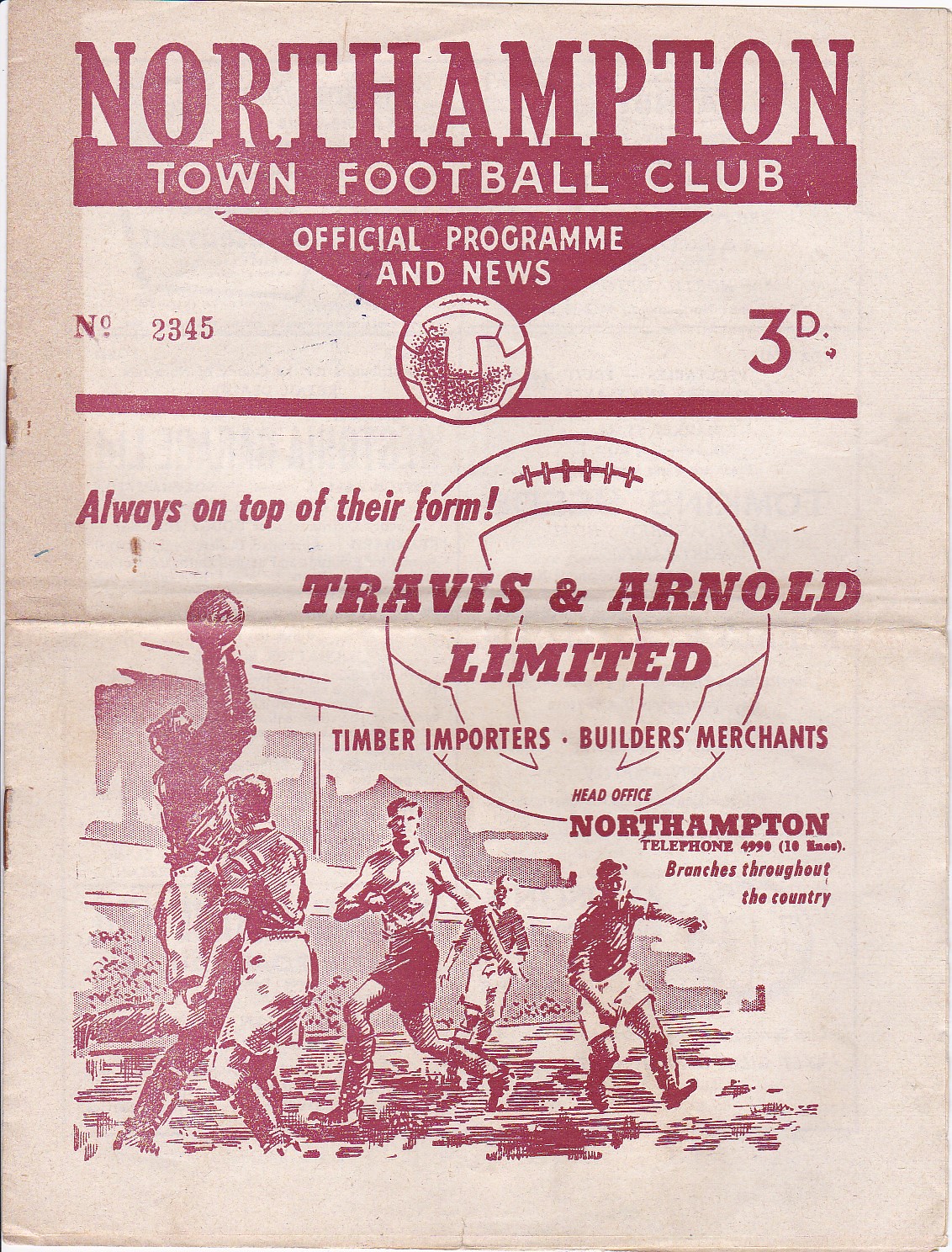The image is the cover of an old magazine, likely an official program for the Northampton Town Football Club. The cover has an off-tan, weathered background with reddish lettering. At the top, bold red text reads "Northampton," underlined by a wide red stripe with white text inside that says "Town Football Club." 

Centered below this header is a downward-pointing red triangle with the words "Official Program and News" in white, and a soccer ball outlined in red at the tip. To the left of the soccer ball, the number 2345 is stamped in red, and to the right, it says "3D". Beneath the soccer ball is a thin red line, slightly overlapped by the ball.

Below this line, a promotional slogan reads "Always on top of their form." Further down, there is a large round image of a soccer ball. Near this image, the text reads "Travis and Arnold Limited, Timber Importers, Builders Merchants, Head Office Northampton," along with the telephone number "4990." Additionally, it mentions "Branches throughout the country." 

To the lower left-hand side of the cover, there is an illustration of five men playing soccer, one of whom appears to be the goalie, either grabbing the ball or preparing to stop it. The overall design reflects its vintage nature with its detailed yet straightforward layout and illustrations.